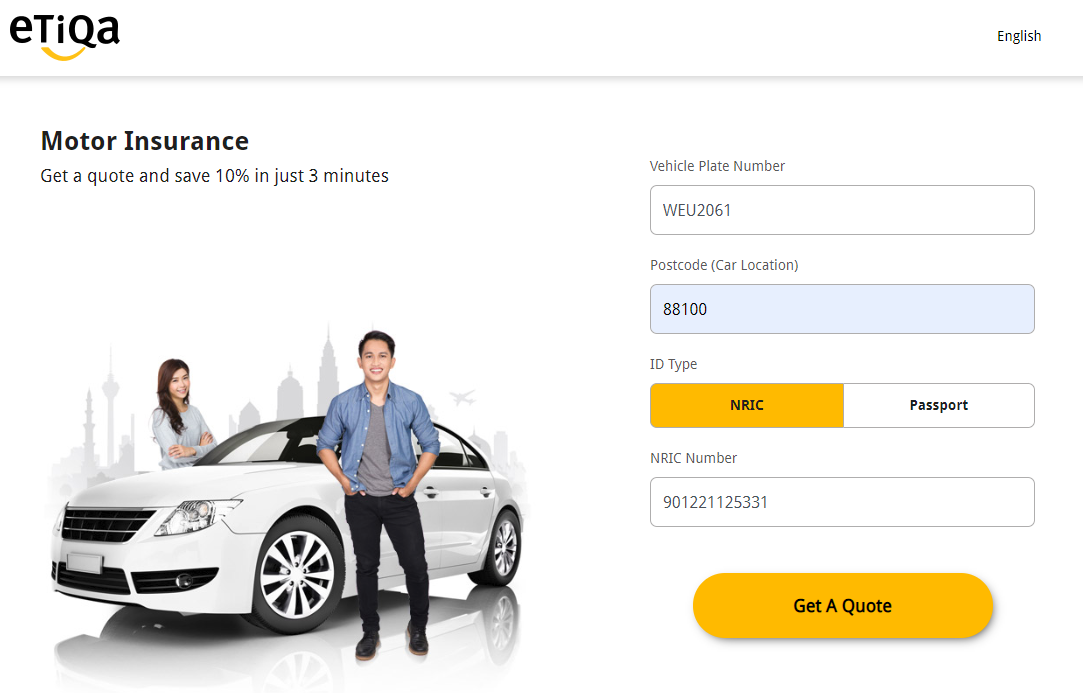Screenshot of the "Etiqa" website, characterized by a clean white background. The top left corner prominently features the site’s logo, "Etiqa," with the "T" and "Q" capitalized and the rest in lowercase, accompanied by a yellow swirl connecting the "T" and "Q." In the upper right corner, a language selection option labeled "English" is visible. Below this, a light gray navigation bar spans the width of the screen.

Dominating the central section of the webpage, a headline reads "Motor Insurance" with a subheading, "Get a quote and save 10% in just 3 minutes," situated in the upper left quadrant. Below this text, there is a graphic depicting an Asian man, presumably in his mid-20s, dressed in a casual outfit consisting of an open denim button-down shirt over a gray t-shirt, paired with black tight pants and black shoes. The man is captured standing with his hands in his pockets, smiling broadly.

The background showcases a highly polished white surface which mirroring a white sedan parked neatly on it. Interestingly, while the car’s reflection is visible, the man’s reflection is absent. In the distance behind the vehicle, an Asian woman wearing a pink shirt is also visible, equally appearing happy.